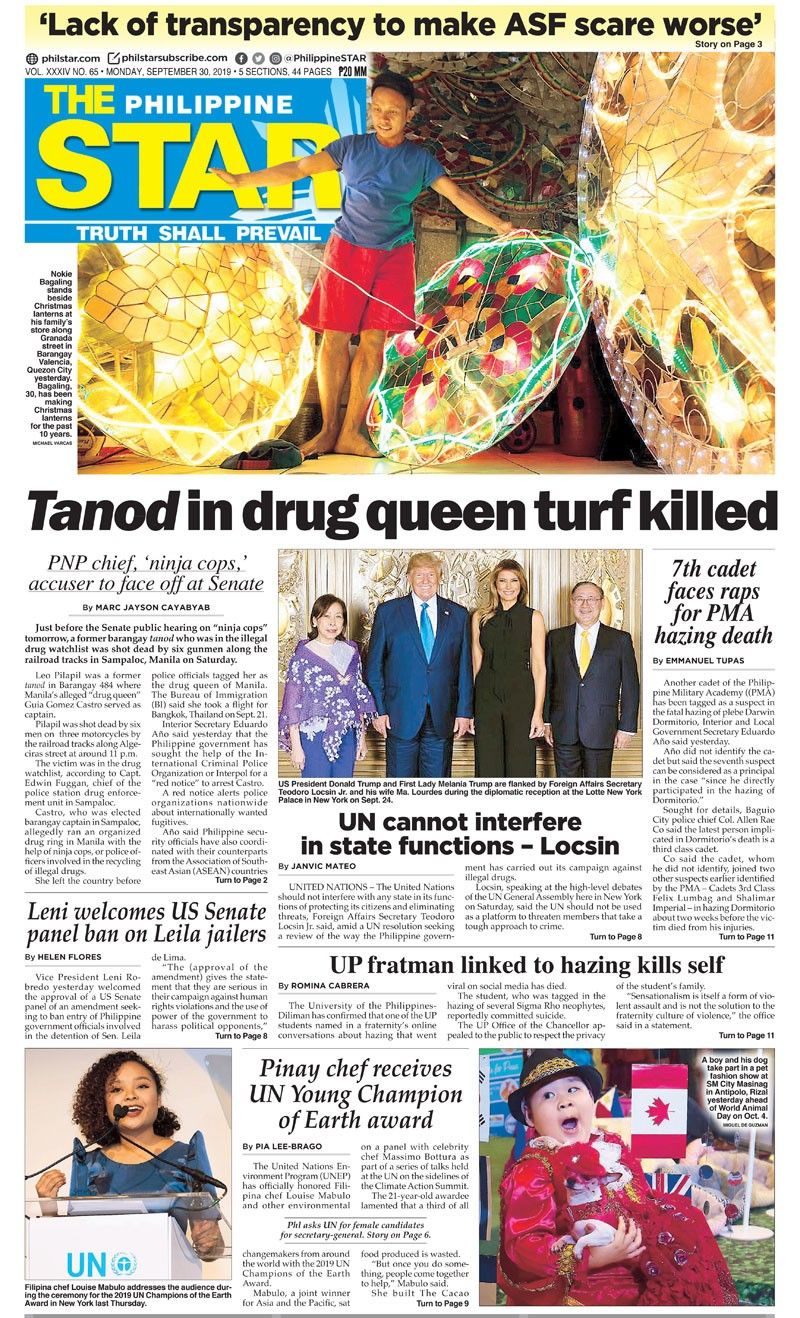This is a detailed description of the front page of the newspaper "The Philippine Star":

---

The front page of "The Philippine Star" highlights several major stories and features a variety of images and headlines. 

At the top of the page, an intriguing headline in bold reads, "Lack of transparency to make ASF scare worse," with further details available on page 3. The newspaper's name, "The Philippine Star," is prominently displayed against a blue background, with its slogan, "Truth shall prevail," printed below it. 

The main photo on the page depicts a man named Bagaling posing next to Christmas lanterns at his family's store along Granada Street in Barangay Valencia, Quezon City. The accompanying caption informs readers that Bagaling, aged 30, has been crafting these lanterns for the past decade, bringing a festive spirit to the community.

Directly below the main photo, a large, striking headline reads, "Tanod and drug queen turf killed. PNP chief, Ninja Cops, accused her to face off at Senate." This reports on a dramatic incident where a former Barangay Tanod, who was listed on the illegal drug watch list, was shot dead by six gunmen along railroad tracks in Sampaloc, Manila. The event has a significant backdrop, as a Senate public hearing on the controversial 'Ninja Cops' is scheduled for the next day.

Adjacent to this, another headline states, "UN cannot function, cannot interfere in state functions," indicating ongoing discussions about the United Nations' role and limitations in state matters.

Adding an international dimension to the front page, there's a prominent photo featuring U.S. President Donald Trump and First Lady Melania Trump. They are seen during a diplomatic reception at the Lotte New York Palace in New York on September 24. The Trumps are flanked by Philippine Foreign Affairs Secretary Teodoro Locsin Jr. and his wife, Ma. Lourdes. The caption highlights the diplomatic engagement between the U.S. and Philippine representatives.

Lastly, on the far side of the page, another headline grabs attention: "Seventh Cadet Faces Raps for PMA Pacing Deaths." This suggests further controversy and legal issues surrounding the Philippine Military Academy.

Overall, the front page of "The Philippine Star" provides a mix of local, national, and international news with detailed images and in-depth captions, reflecting significant events impacting both the Philippines and the world.